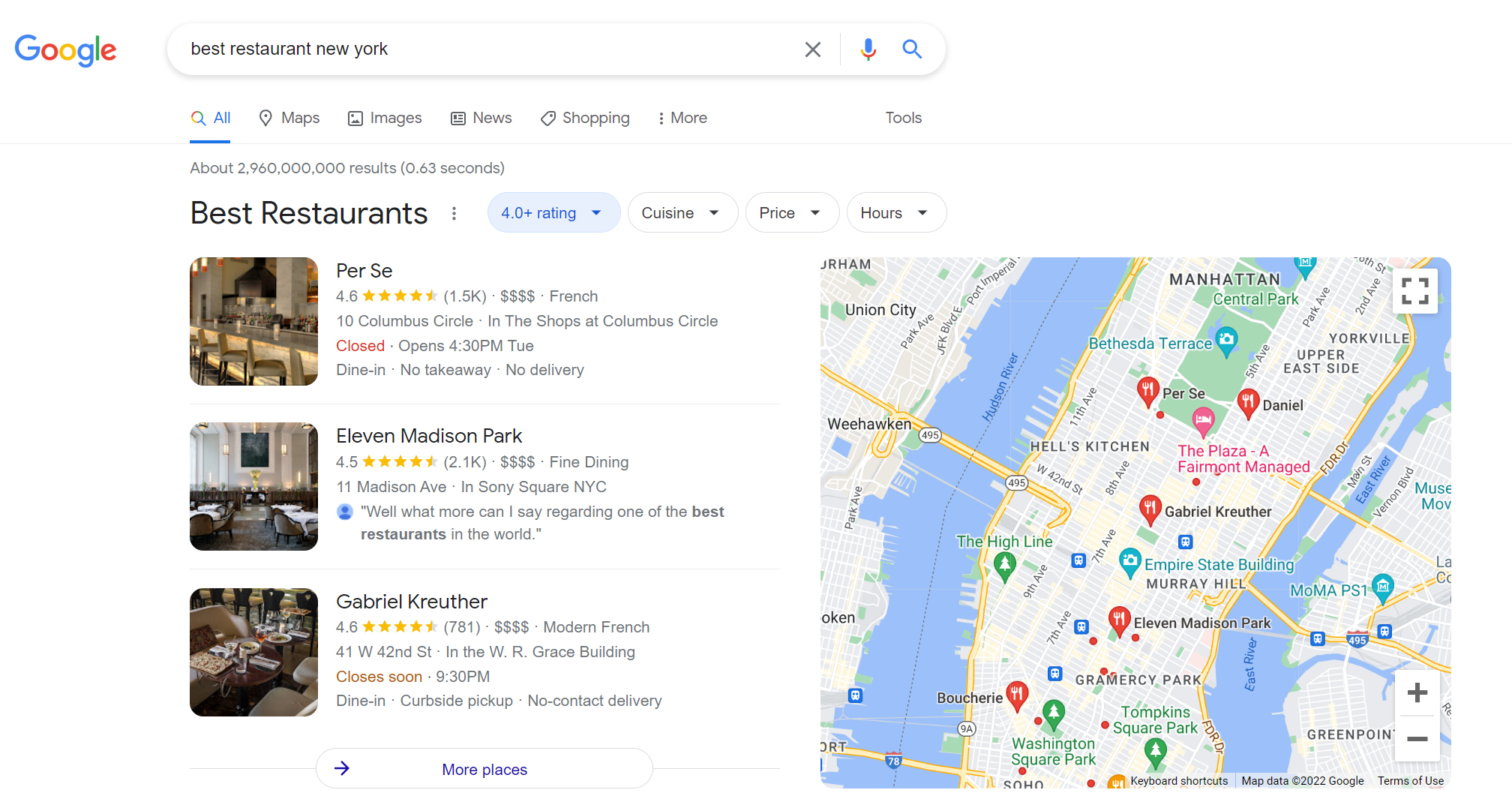The image depicts a search engine results page for the query "best restaurants in New York." In the search field, the query is entered visibly, with an "X" icon, a microphone icon, and a magnifying glass icon located in the upper right corner of the field. Below the search bar, the standard menu options are present, including "All," "Maps," "Images," "News," "Shopping," "More," and "Tools."

The results summarize that there are approximately 292 billion 960 million possibilities, retrieved in just 0.263 seconds. The list of results begins with "Per Se," noted as temporarily closed, and its location is specified as Time Warner Center, 10 Columbus Circle, New York City. The second result is "Eleven Madison Park," located at 11 Madison Avenue, New York City.